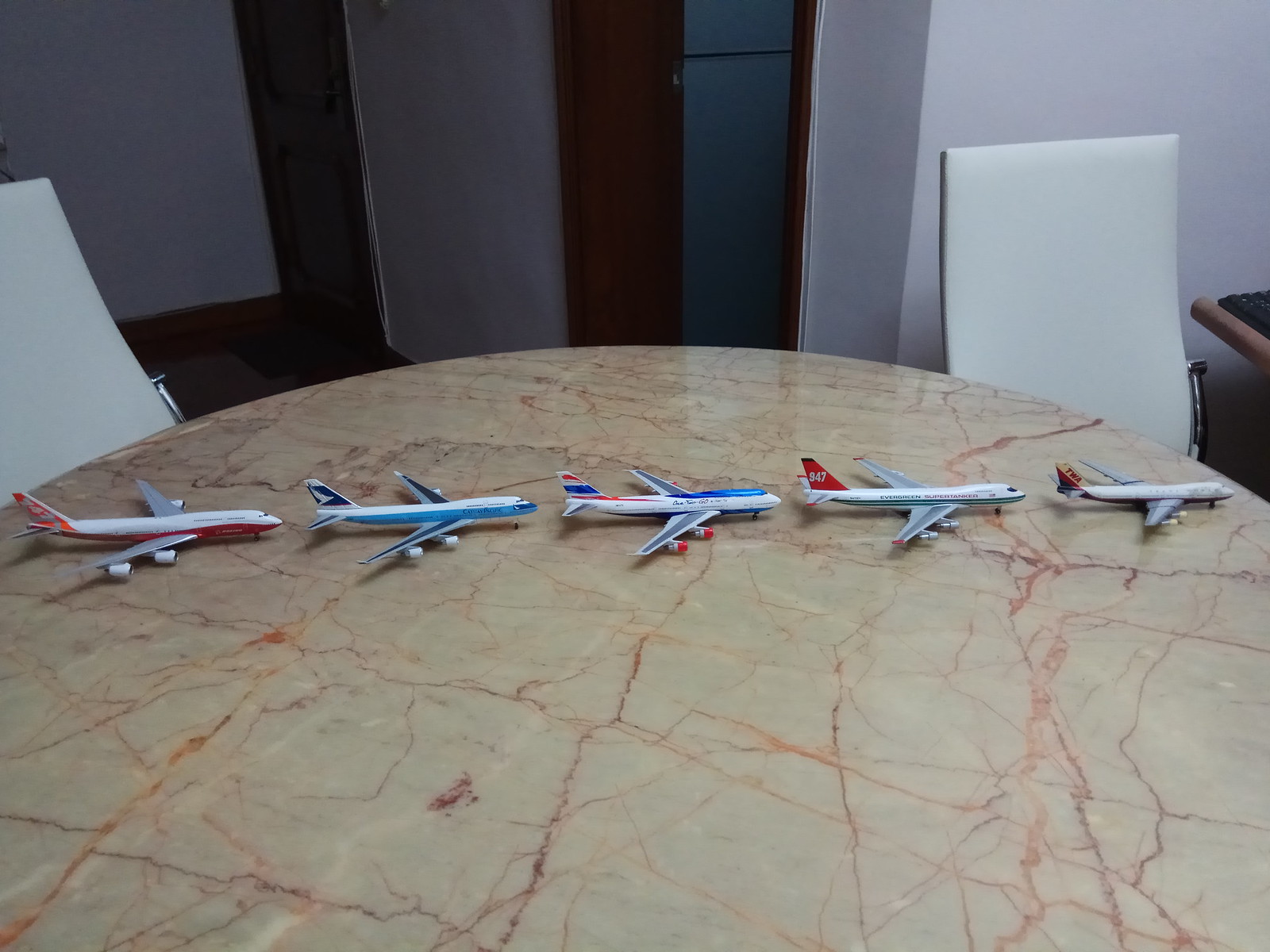In the photograph, a round dining table with a cream-white marble countertop, accentuated with brown design lines, holds five toy airplanes meticulously lined up from left to right. The planes, varying in design and color, are all oriented towards the right side of the image. The first plane is small and white, followed by a slightly larger white plane. The third plane features a double-deck design adorned in blue, white, and red colors. The fourth plane, with blue and white hues, represents the Cathay Pacific brand, while the fifth is a Boeing 747 with gray and red accents. This table is surrounded by two dining chairs on either side, both white with silver metal frames. In the background, the living room setting is delineated by white walls, two dark brown wooden doors, and visible alleyways.